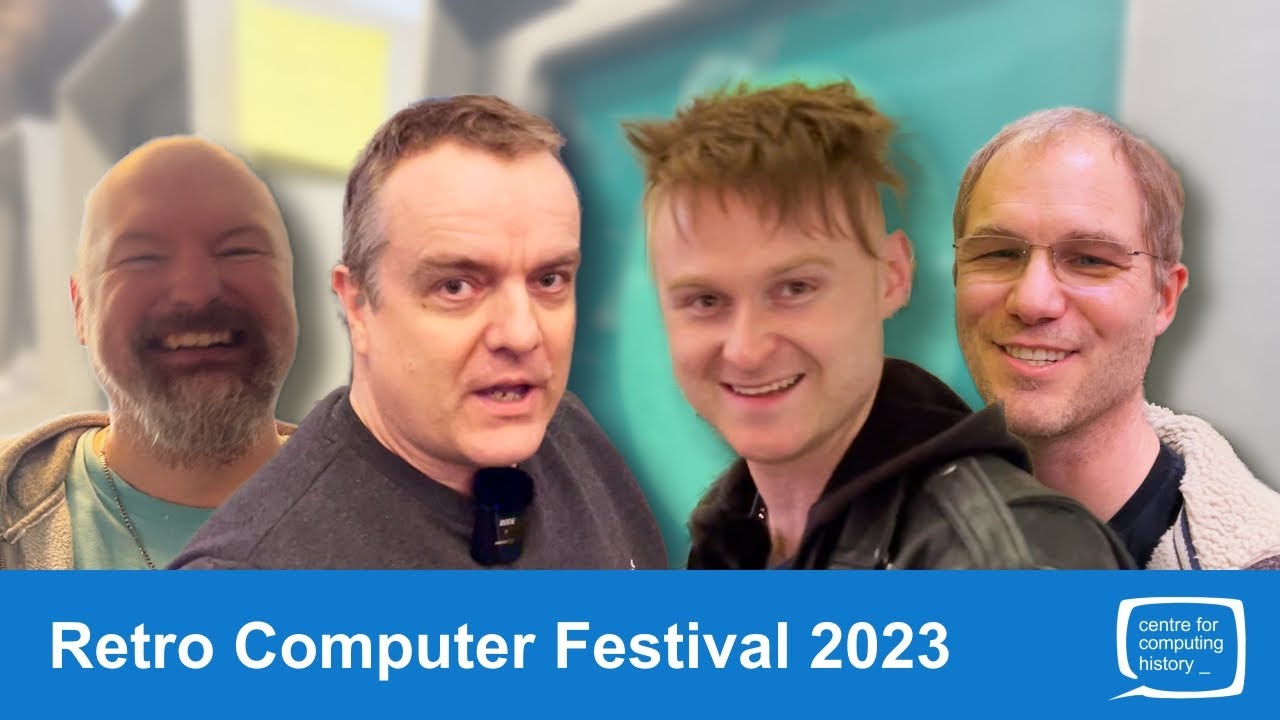This image appears to be a promotional poster or webpage for the "Retro Computer Festival 2023," organized by the Center for Computing History. The design features a distinctive blue banner running along the bottom, prominently displaying the event's name. A white TV icon is positioned on the right side of the banner. Above this banner, the central portion of the graphic showcases four photos of white men, seemingly photoshopped in front of an indeterminate background that resembles an office building.

From left to right, the first man is bald with a beard and is smiling broadly. He is wearing a blue shirt, a sweater, and a necklace. The second man has thin, grayish hair and is caught mid-speech; he wears a black or gray sweater with a peculiar collar detail. The third man has scruffy hair and a jacket, his expression also a smile while he looks at the camera. The fourth man has a receding hairline, glasses, and is sporting a black shirt with a jacket; he, too, is smiling pleasantly. This composite effectively captures the essence and personalities of the festival's participants.